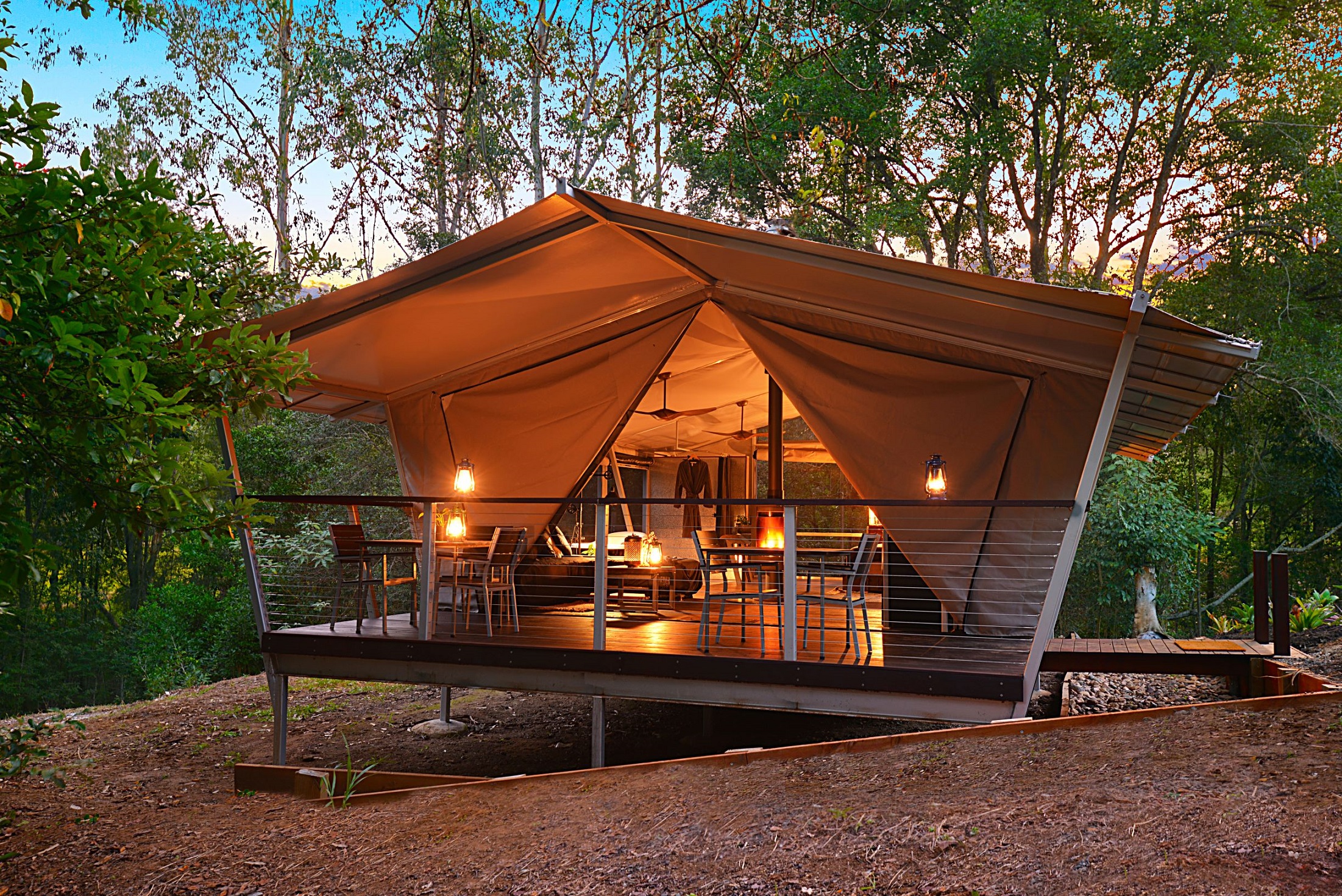The image captures an elevated platform structure amidst a lightly dense forest, shrouded by a high-quality brown canvas tent. This elaborate, modern tent, resembling a cabin, stands firm on long metal poles to prevent flooding. Accessible via a small bridge-like walkway, the platform features dark wood paneling and is surrounded by lush greenery and tall trees under a blue, cloud-dappled sky. Orange lanterns dot the surroundings, adding a warm glow.

Inside the tent, the front flaps are pinned back, revealing a well-lit interior adorned with numerous tables, chairs, and other furnishings, including a couch and coffee table. A wood-burning stove with a central pipe is prominent, accompanied by fans and electrical power, suggesting significant amenities. A dress-like object hangs in the back, barely visible. The scene is free of people, highlighting a serene, well-equipped spot perfect for relaxation or possibly a high-end glamping experience.